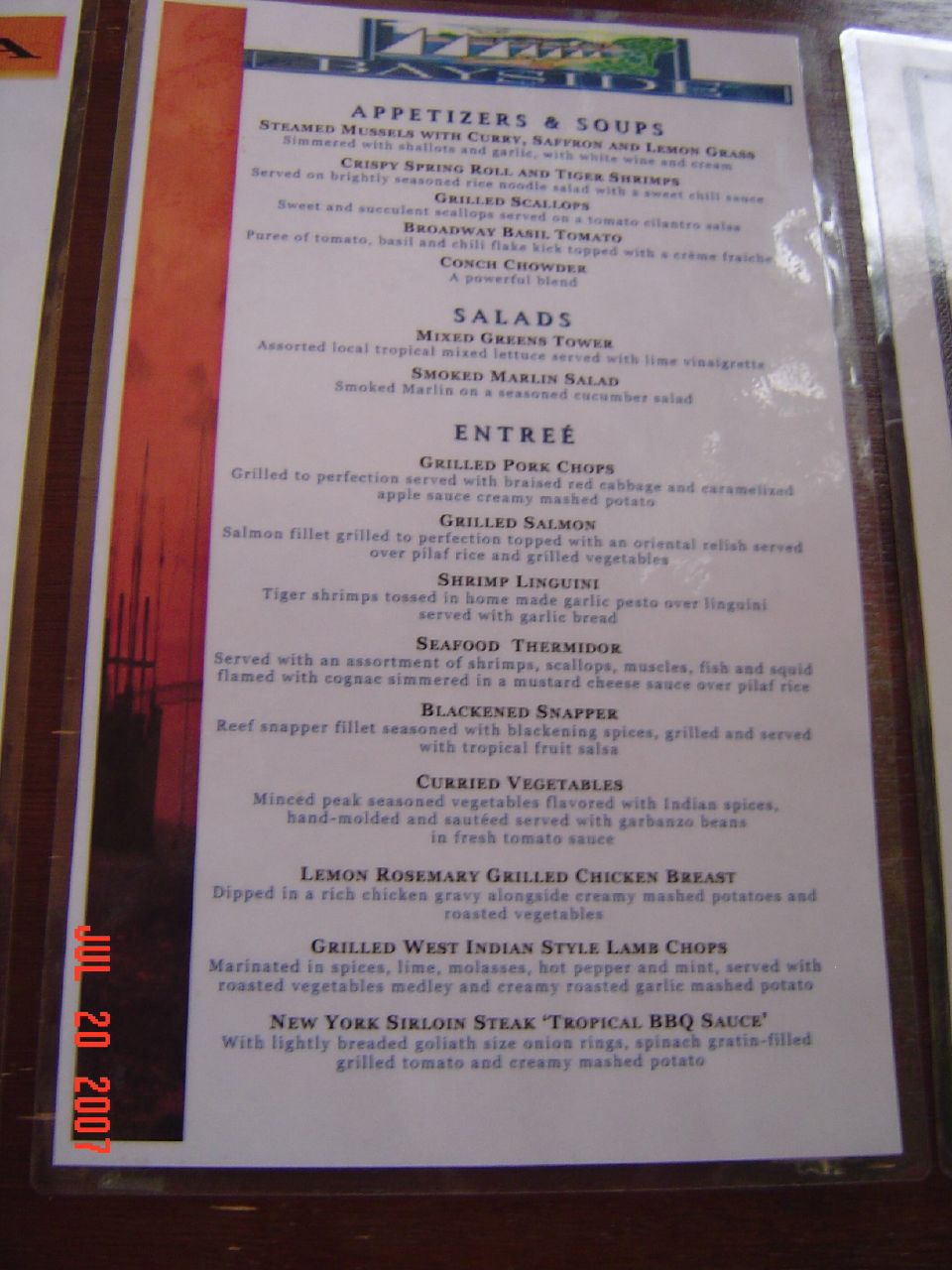The image appears to be a photograph taken with a digital camera, as evidenced by the bright orange timestamp in the bottom left corner, displaying the date "JUL 20 2007" in an analog-style, all-caps font. The focus of the photograph is a laminated menu from a restaurant named "Bayside." The top of the menu features the word "BAYSIDE" alongside a logo depicting a body of water and white sailboats, evoking a nautical theme.

Organized into clearly defined sections, the menu includes headings like "APPETIZERS AND SOUPS" in a bold, blue all-caps font. Below this heading, there are subcategories such as "SALADS" and "ENTRÉES." Each food item is listed in black, all-caps lettering, with detailed descriptions in a standard mixture of uppercase and lowercase letters in a dark blue font. These descriptions outline the ingredients and components of each dish, providing potential diners with a comprehensive understanding of the menu offerings.